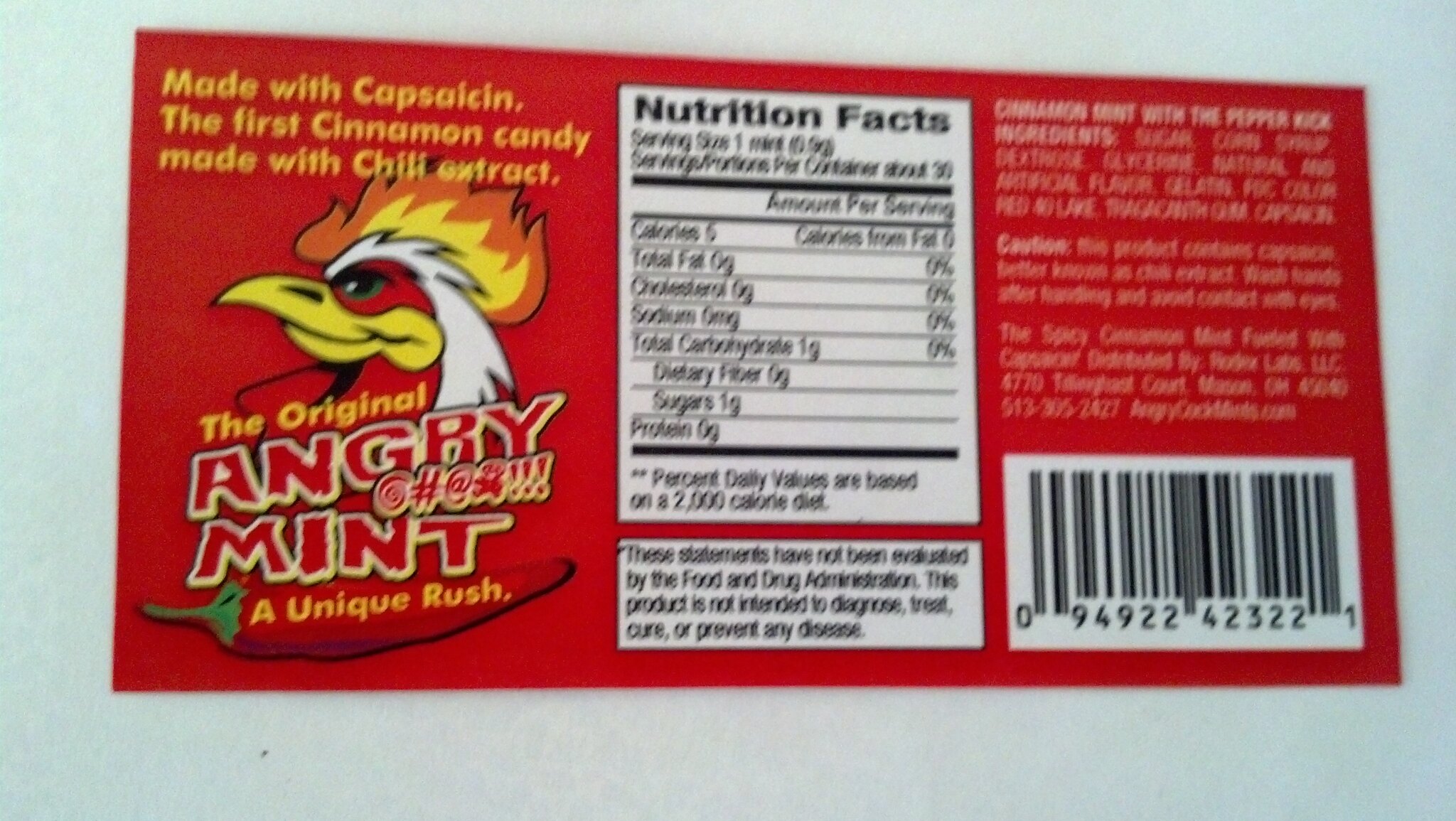This is a detailed photograph of a candy package showcasing a unique spicy snack. The package is predominantly red with vibrant yellow text that announces its distinctive nature—this is the first cinnamon candy made with chili extract. Central to the design is the company logo, featuring a white chicken or rooster with a yellow bill and red markings on its face. Notably, the rooster has a plume of flame instead of a typical comb, emphasizing the candy's fiery theme. Below the logo, bold text proclaims "The Original Angry Mint," with some abstract swearing symbols adding to the aggressive branding. Further down, there's the phrase "A Unique Rush," displayed in yellow text over an image of a red chili with a green stem. 

On the right side of the package, the nutritional facts are displayed in a white rectangle with black text, detailing calories, total fat, sodium, and other nutritional information. The ingredients list is also presented in a similar white box beneath the nutritional facts. A caution section and a barcode, complete with white text above the barcode, are placed at the bottom right corner of the package. This candy promises a hot and spicy experience, combining the heat of chili with the sweet spice of cinnamon.